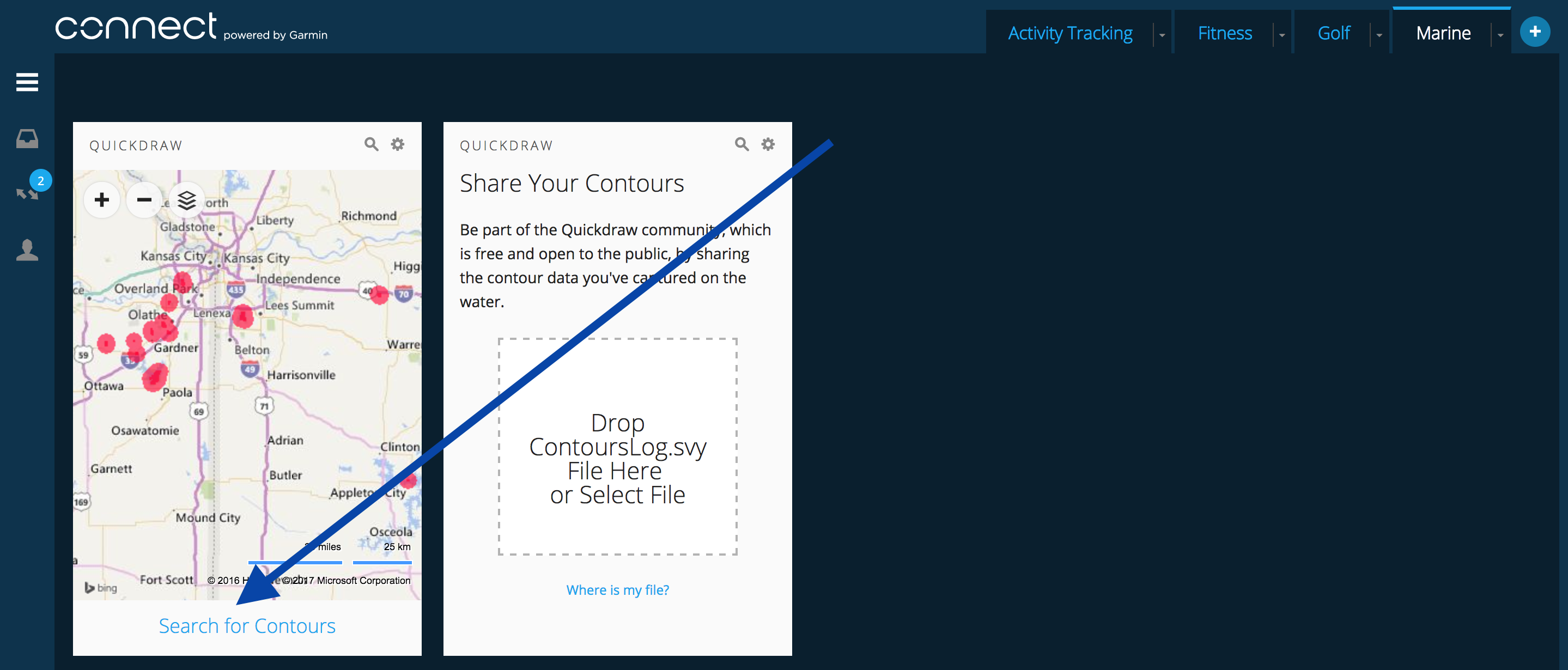The screenshot from the Garmin Connect platform showcases a spacious, dark navy interface with several features related to maps and GPS data. Dominating the screen, one image depicts an overview map of Kansas City with numerous areas marked in red, though the specific purpose of these markings is not detailed. At the bottom of this map, a prominent button labeled "Search for Contours" invites user interaction.

Adjacent to this, another section highlights a feature titled "Share Your Contours." This interactive area allows users to drag and drop files to contribute to the Quick Draw Community. The community is described as a free and public resource for sharing contour data captured on water, with a defined space edged in dotted lines for easy file upload, presumably for elevation data acquired via mobile devices.